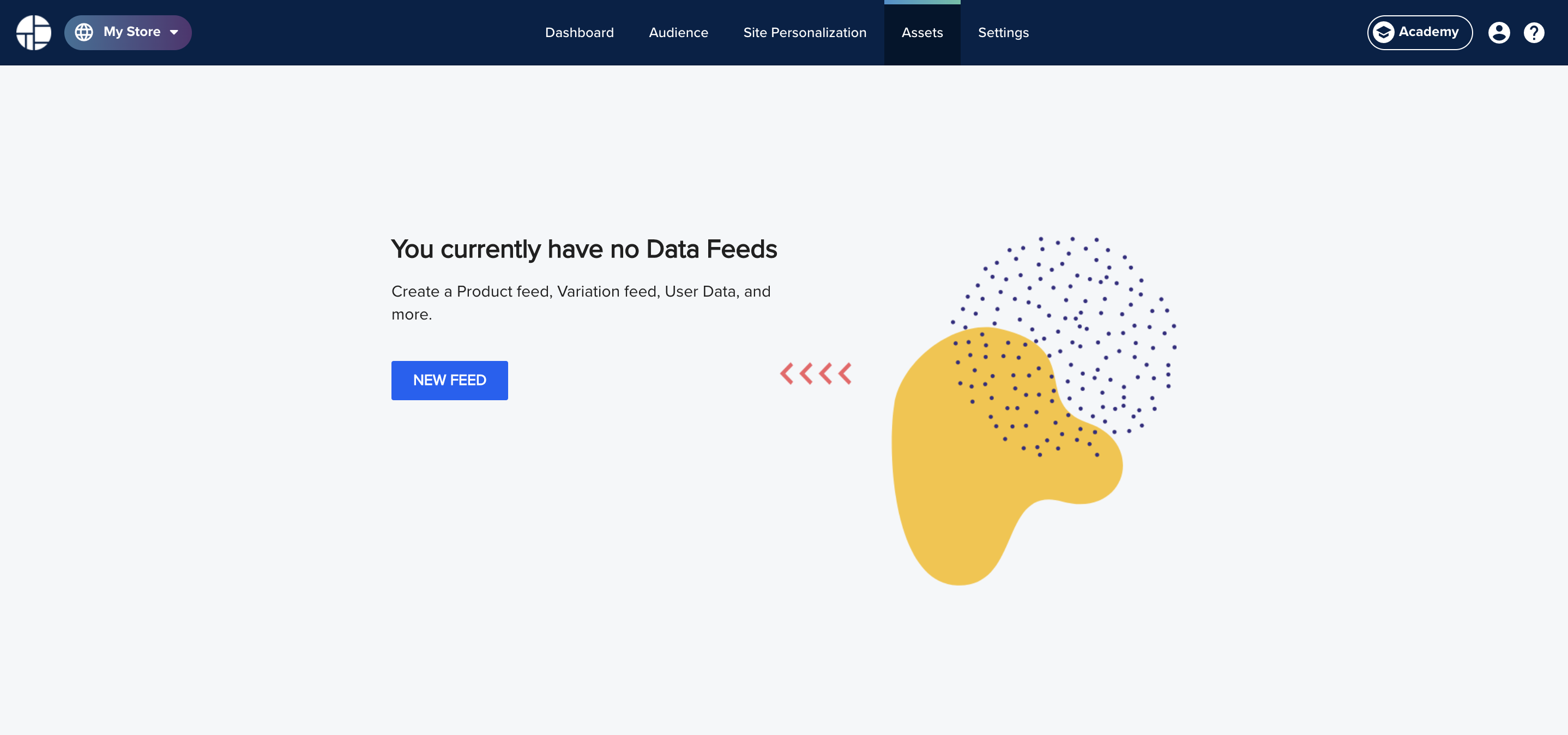The image depicts a webpage from an unspecified website. At the very top of the page is a prominent blue header bar. Located in the upper left corner of the header is a drop-down menu labeled "My Store." Adjacent to this are five navigation options arranged from left to right: Dashboard, Audience, Site Personalization, Assets, and Settings. The "Assets" tab is currently selected. To the right of these navigation options is an "Academy" button, along with an account button and a help button marked with a question mark.

The main section of the "Assets" page features a primarily grayish-white background. Centrally positioned is the message "You currently have no data feeds. Create a product feed, variation feed, user data, and more." Below this message is a clickable blue button labeled "News Feed." To the right of the textual information is a dynamic animation composed of amorphous, colorful elements: a yellow blob, superimposed with blue dots forming a circular pattern, and four red arrows pointing to the left.